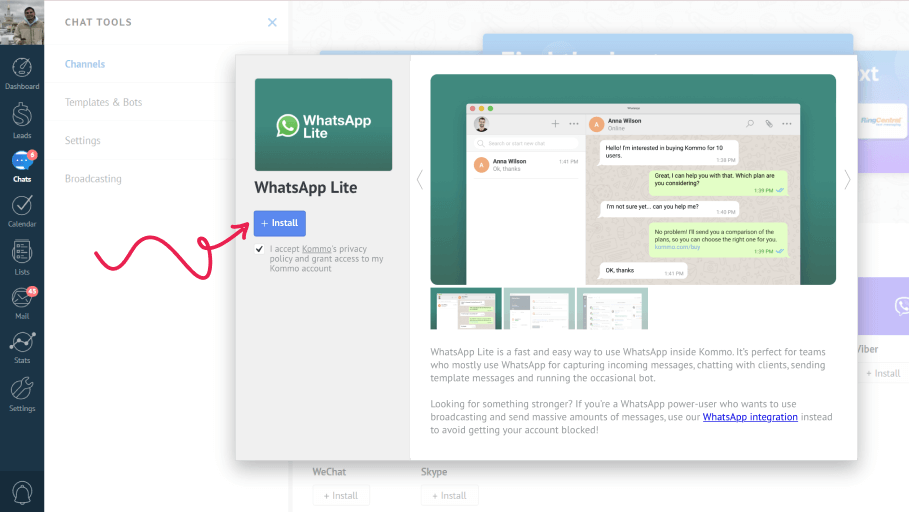A screenshot of a website dedicated to chat tools is displayed. The site features a vertical menu on the left-hand side, listing options such as Dashboard, Leads, Chats, Calendar, Links, and Mail. The 'Chats' option is currently highlighted, indicating that this page is active. Within the main Chat Tools section of the page, several subcategories are visible, including Channels, Templates, Settings, and Broadcasting. The 'Channels' subcategory is selected, as denoted by its blue highlight. A pop-up box appears prominently on the screen for selecting a channel type. The upper left corner of this box identifies the channel as "WhatsApp Lite," with 'Lite' explicitly spelled out as L-I-T-E. A squiggly red arrow directs attention to an 'Install' button, suggesting the option to install the Lite version of WhatsApp on the computer. The main body of the pop-up box includes an image depicting the WhatsApp Lite interface and accompanying text that describes the application's functionalities.